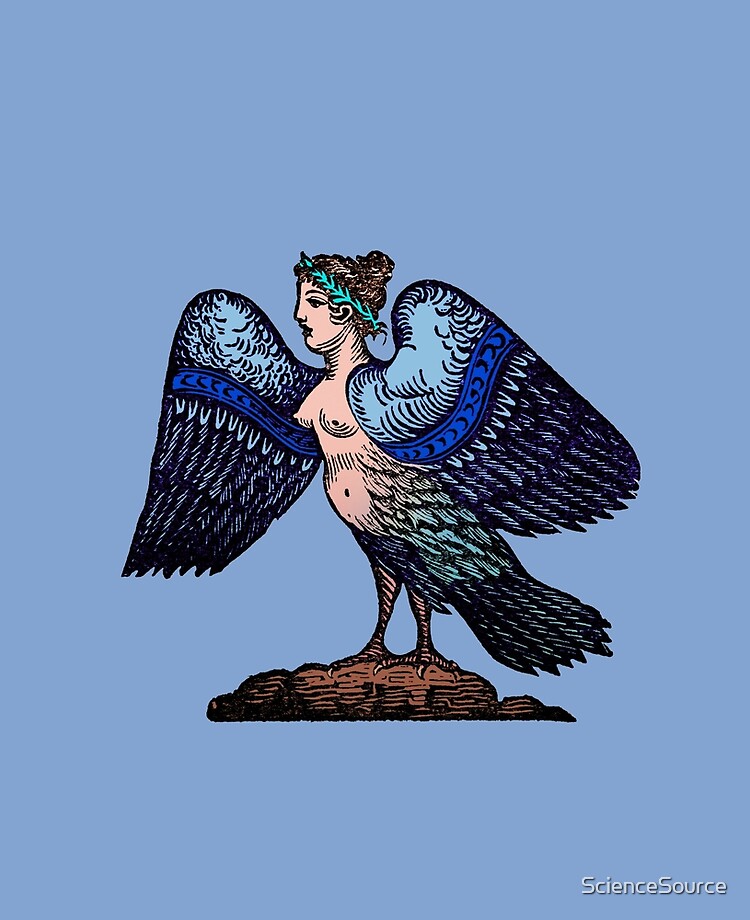This detailed illustration depicts a harpy, a mythological creature with the upper body of a woman and the lower body of a bird, standing on rocky terrain. The harpy, resembling an eagle, features light blue wings, a light blue tail, and bird-like feet. Her upper body is human, with visible breasts and hair tied up, adorned with a light green laurel. The background of the image is a solid light blue, enhancing the vibrant colors of the harpy, which include various shades of blue, green, brown, beige, and white. Positioned in the middle of the artwork is the harpy itself, while the text "science source" is located in the lower right corner, indicating the source of the illustration. This piece effectively blends the avian and human elements, showcasing the artistry involved in creating such a captivating hybrid creature.